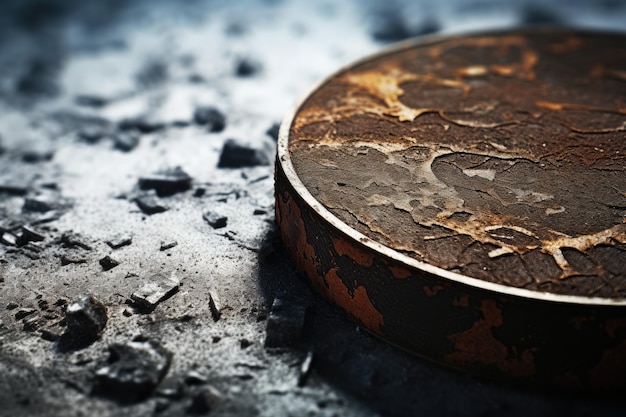This photograph depicts the floor of an abandoned building, showcasing a large, heavily rusted circular metal object positioned on the right side. This object, likely made of iron, has a corroded surface marked with vast patches of brown and reddish rust. Surrounding this central piece is a forged iron ring, and inside, the metal is extensively rusted. 

To the left of the circular object, scattered across the ground, are various smaller metal shards and what appears to be debris. These smaller pieces are predominantly gray or silver, though some show signs of rust as well. Additionally, there are shards that resemble black glass, adding to the chaotic scene of decay. The ground itself may be concrete, indicative of the structural flooring of the abandoned site. 

There is a light source visible in the background, shining through and illuminating parts of the scene, but it remains out of focus. No text or lettering is present in the photograph, leaving the objects and their condition as the primary subjects of interest. The image captures a moment of industrial ruin, detailing the textures and decay of metal left to deteriorate over time.